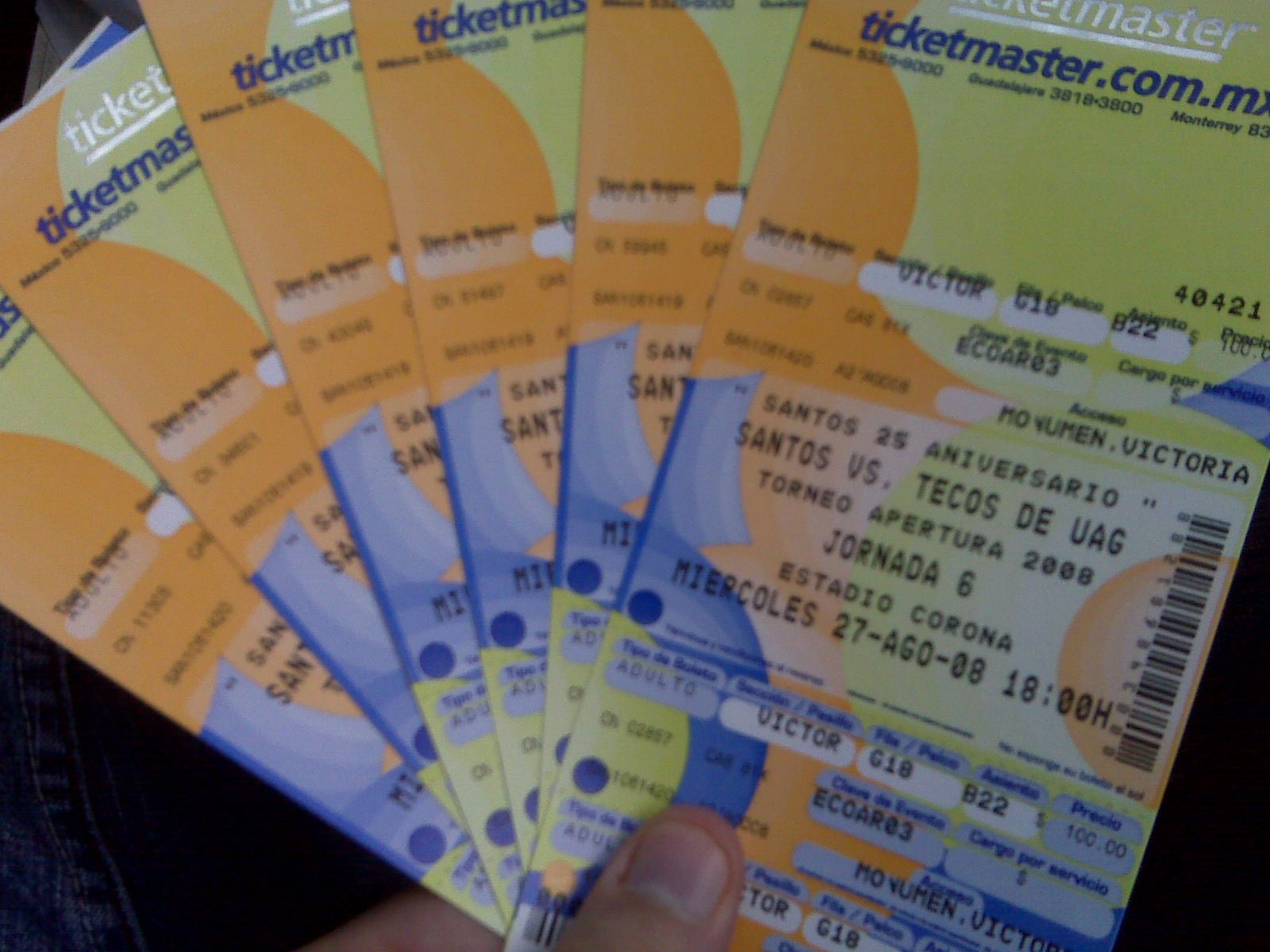In the image, someone is holding six fanned-out Ticketmaster tickets over their lap, with their thumb and forefinger gripping the tickets at the bottom. The tickets are a mix of green, orange, blue, and white, featuring black text detailing the event, which appears to be written in Spanish. Although the top and sides of the tickets are slightly cut off, notable details include the Ticketmaster logo in shiny silver at the top, followed by a blue URL for ticketmaster.com. The text mentions the event "Santos 25th Anniversario" between "Santos vs. Tecos DeUAG," set for "Jornada 6" at "Estadio Corona," occurring on "27 AGO 08" at "18:00." Other details such as seat numbers "Victor G-18" and "V-22," a price of "$100," and a barcode can also be seen. The tickets, held over blue jeans, provide clear information about seating, date, time, and venue.